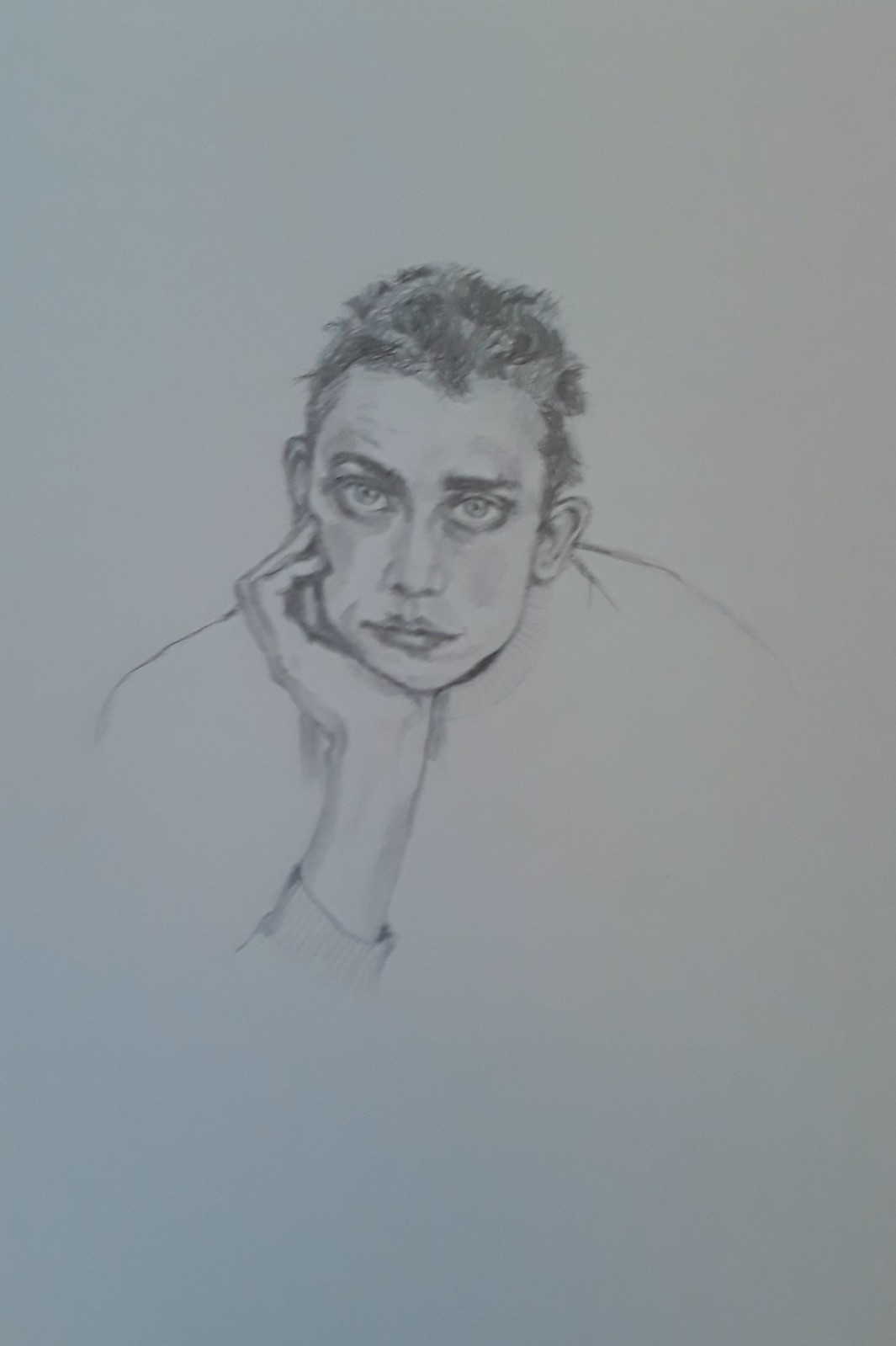The artwork is a charcoal drawing of an androgynous person rendered on a medium gray background. The subject features short, spiky hair that is cropped shorter on the sides and left slightly longer on top. They possess large, dark, and well-defined eyebrows above their expressive eyes, which are accentuated by rings suggesting smudged makeup, hinting at recent tears. The person's chin rests thoughtfully in their hand. Skillful shading conveys a sense of color in their cheeks and just above their eyebrows, enhancing the dimensionality of their well-shaped nose and full, neutral lips. Their attire includes a long-sleeved shirt, contributing to the overall contemplative mood of the piece.